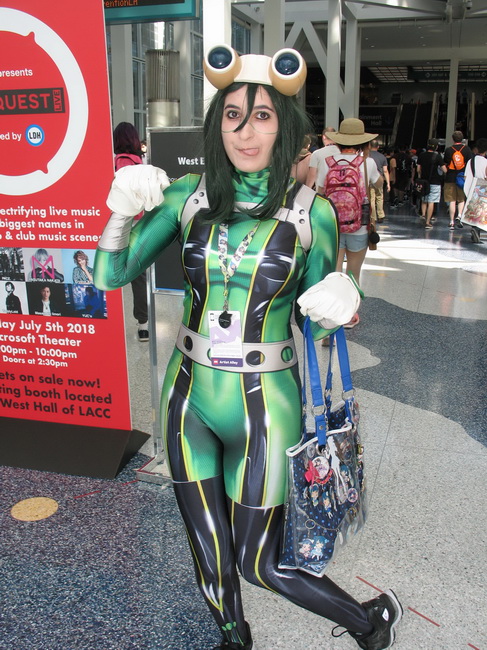In this photographic image set inside an expo hall, a young white woman, likely in her teens or twenties, strikes a playful pose, lifting one leg slightly and sticking out her tongue. She is dressed in a vibrant green, form-fitting superhero costume adorned with black leather stripes running down the chest and legs, complemented by black boots. Her long black hair flows freely, and she wears a distinctive headband featuring two lens-like structures resembling bug eyes or binoculars. On her hands are black gloves, though one account mentioned white gloves, the black gloves detail is more predominant. She carries a reusable shopping bag, adorned with anime character designs, adding a touch of personal flair to her attire.

In the background, various people move through the hall; one person is seen walking away while wearing a brown hat, blue shorts, and a red backpack. Several women are heading towards a doorway. A partially visible red poster to her left reads about an electrifying live music event featuring the biggest names in the club scene, scheduled for July 5th, 2018, at a specific theater with tickets available at the west hall of the LACC. The floor appears to be gray granite, and the setting includes prominent lighting and structural pillars, indicating a likely convention or cosplay event atmosphere.